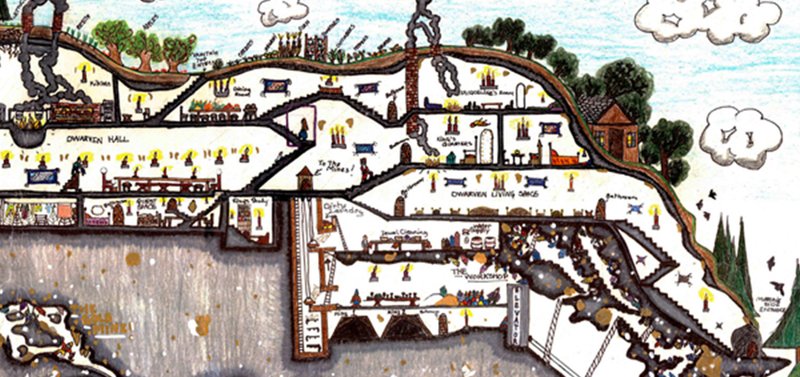This captivating horizontal painting vividly illustrates a whimsical cutout of a living area built into the side of a mountain. The top of the image features a picturesque blue sky dotted with fluffy white clouds, trees of various colors, and grass creating a roller coaster-like pattern from left to right. Nestled on the hillside is a charming brown house, accompanied by birds soaring in the sky. The focal point, however, is the intricate depiction of the mountain's interior, resembling an elaborate ant hill cross-section with various interconnected rooms in diverse shapes and sizes, bordered in black. The interior is primarily white, accentuated with hues of blue, brown, gray, and yellow, giving it a lively feel. 

This underground city unfolds over six distinct levels, filled with around 20 to 25 rooms. These spaces buzz with activity: people sit at tables, navigate black and brown staircases, and engage in daily chores. Certain rooms suggest living areas, complete with beds and possibly laundry rooms, while others appear to be dedicated to various work activities. The detail is striking yet simple, evoking an imaginative, almost stick-figure-like charm. This whimsical and richly detailed painting invites viewers to explore its miniature world brimming with life and curiosity.